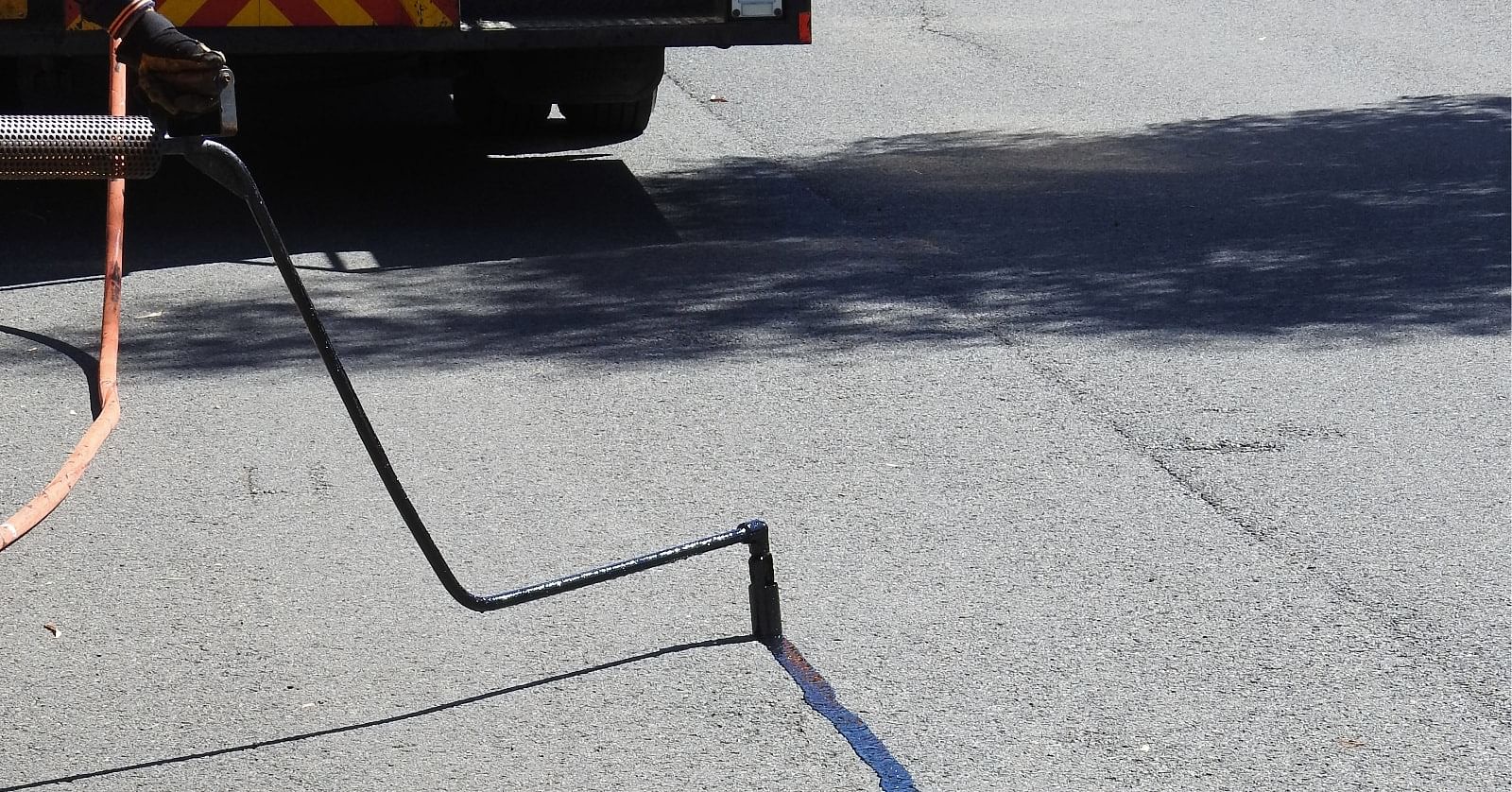In this image, we see a grey roadway stretching ahead. Prominently positioned in the scene is a truck adorned with diagonal orange and yellow stripes. The truck’s black wheels are partially visible, obscured by shadows. On the right side of the image, the shadow of a tree suggests the presence of a tree just outside the frame. Sunlight appears to illuminate the scene from that direction, casting sharp shadows.

A distinguishing feature of the truck is a black L-shaped pipe extending from it, reaching down to the road's surface. This pipe seems to be dispensing a bluish substance, creating a watermark-like stain on the asphalt. Additionally, an orange hose trails behind the truck, hinting that the vehicle might be engaged in a roadway marking or maintenance activity. The blue stain left on the road could potentially be indicative of some sort of spray paint marker or similar substance used in roadworks.